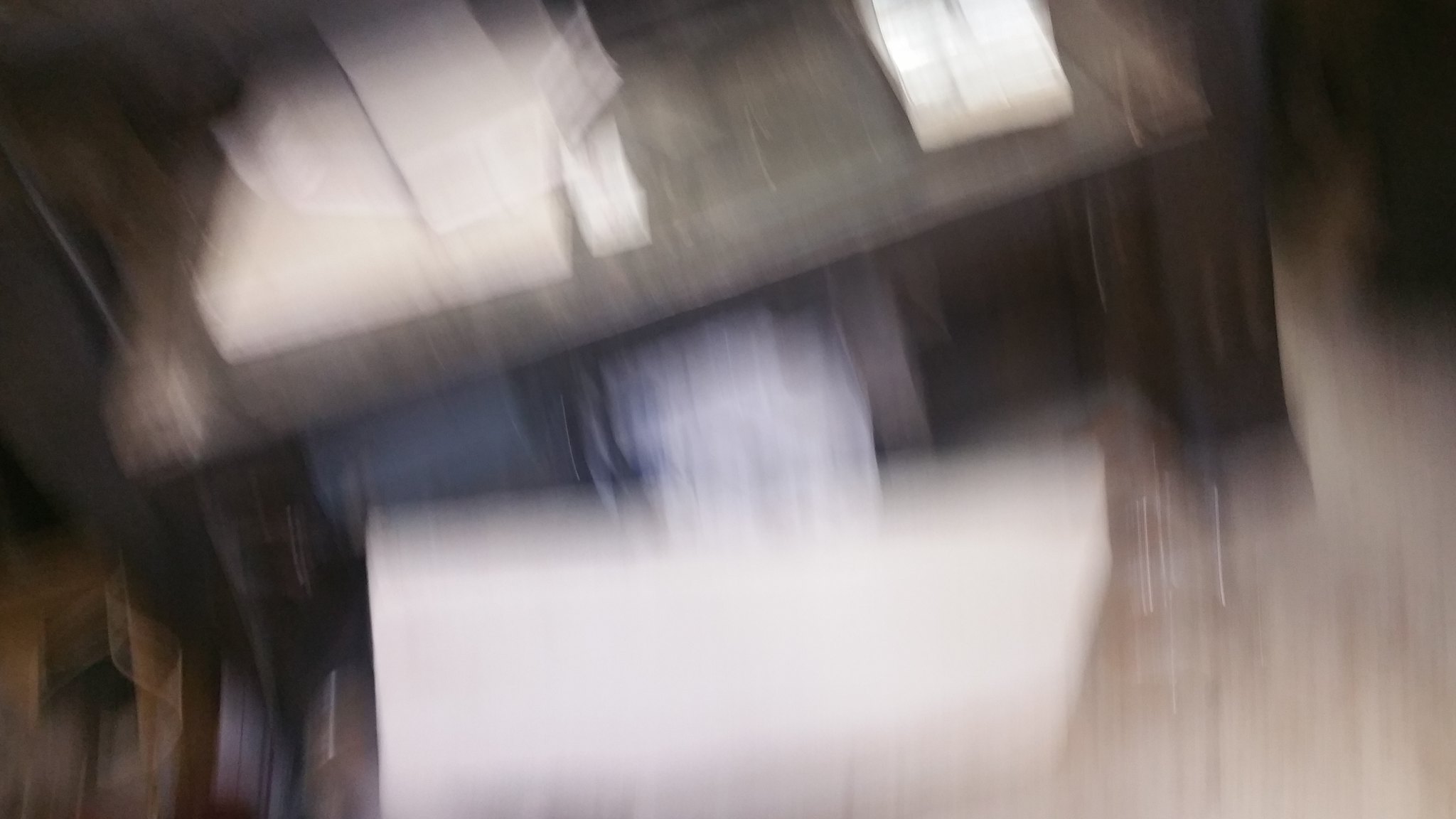The image is highly blurry, making identification challenging. It appears to feature a light tan surface, possibly a table, on which a black unit resembling a small home printer is placed. The printer-like object is topped with several white rectangular boxes, and there is another white item positioned to its right. Additionally, a piece of computer paper seems to be protruding from the side of the unit. However, the exact point of exit for the paper is unclear. There is a narrow white opening in the center of the unit's front, which could potentially be a paper slot, though its precise function is ambiguous.